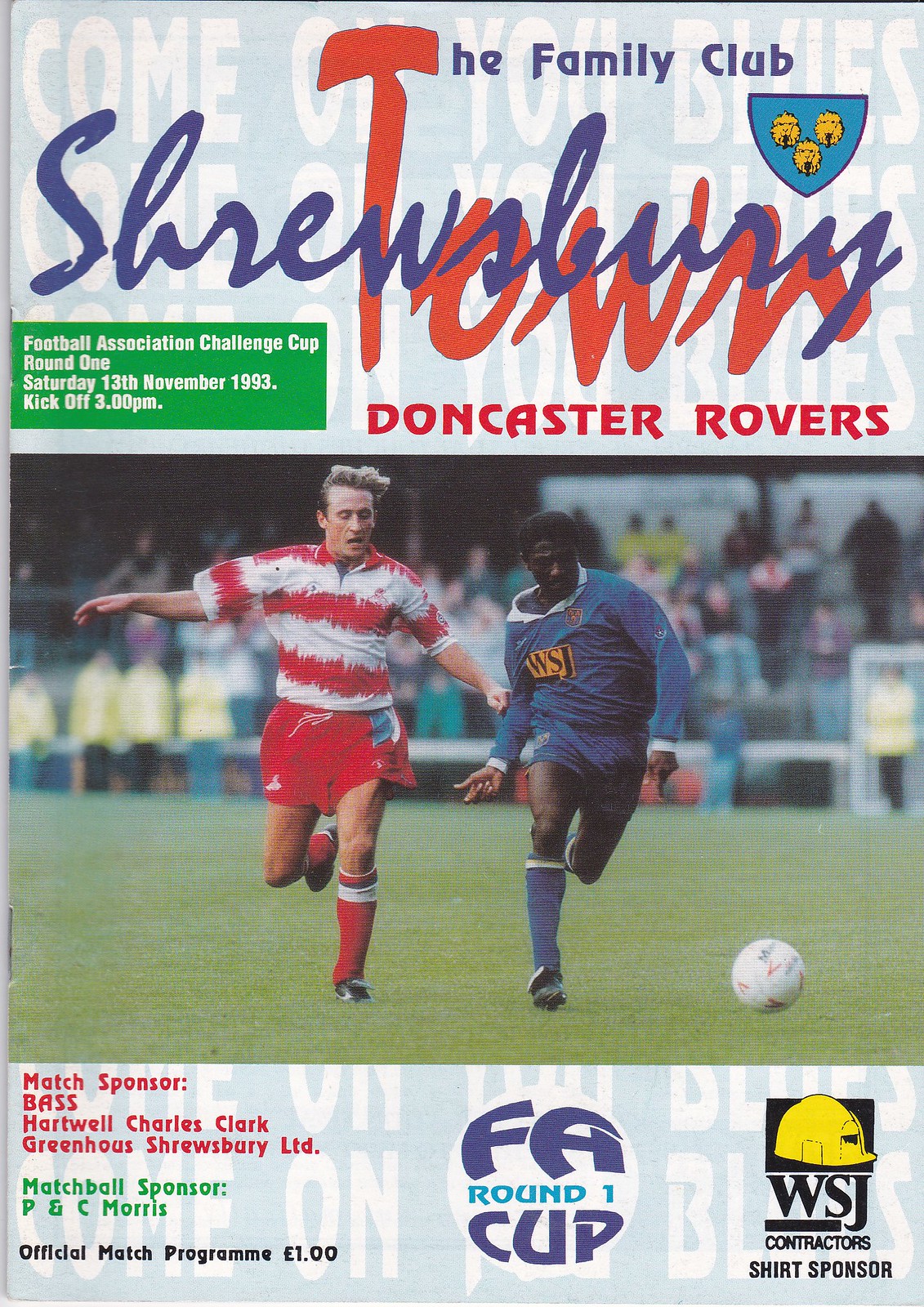This photographic image captures the front cover of a soccer program for the Football Association (FA) Challenge Cup Round 1 match between Shrewsbury Town and Doncaster Rovers, held on Saturday, 13th of November, 1993, with kick-off at 3 p.m. The cover features a dynamic action shot of two soccer players: a white man in a red and white striped jersey with white shorts, complemented by red and white socks, and a black man in a blue jersey adorned with an orange logo, paired with blue shorts, blue socks, and black sneakers. Both players are intensely focused as they chase a white soccer ball. The background subtly shows the blurred image of stands filled with spectators.

Positioned at the bottom of the cover in a green box are several sponsor details: "Match Sponsor: Bass, Hartwell Charles Clark, Greenhouse Shrewsbury Limited," "Match Ball Sponsor: PNC Morris," and "Official Match Program: One Pound." Centered within this box are the words "FA Round 1 Cup," flanked to the right by an image of a yellow construction hat labeled "WSJ Contractors" and the text "Shirt Sponsor."

In the upper right-hand corner, there’s a logo with shields and text that reads, "The Family Club, Shrewsbury Town, Doncaster Rovers, Football Association Challenge Cup, Round 1." The background of the cover repeats the phrase "Come on You Blues" in light blue, reinforcing Shrewsbury Town’s team spirit.